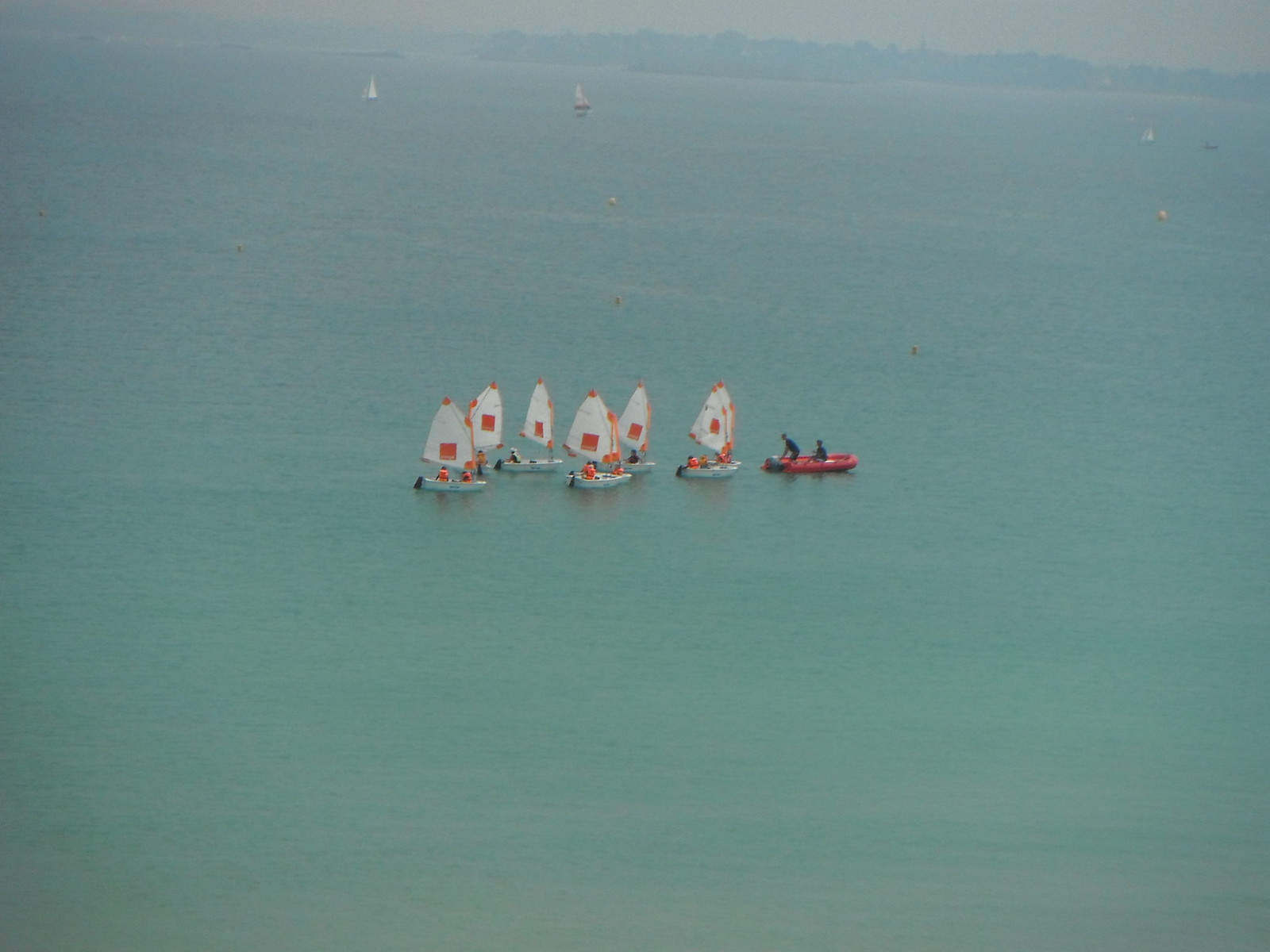This aerial photograph captures a serene scene on a vast, calm body of water, possibly the ocean, characterized by its greenish-blue hue. Six small sailboats dot the center of the image, each adorned with white triangular sails featuring a distinctive red square in the middle. The boats themselves are white, with a sharp-edged rectangular shape, and are manned by people wearing bright safety orange outfits, likely life jackets. The individuals aboard the sailboats are small and barely discernable, emphasizing the distant perspective of the shot. To the right of the sailboats, a red inflatable raft with two people dressed in black is visible, one of whom appears to be operating a motor at the back. The photograph, taken during the day, has a hazy, smoggy background that slightly obscures the distant coastline and tree line at the top of the image. The water remains calm, with no noticeable waves or ripples, completing the tranquil and somewhat ethereal atmosphere of the scene.